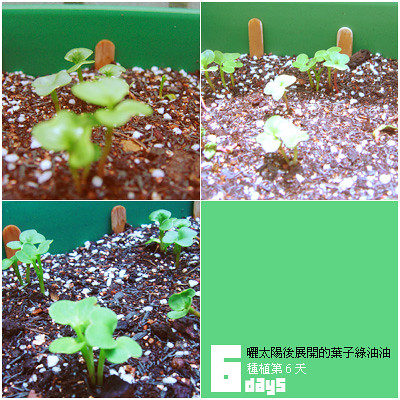The image is a collage of four sections, capturing the growth of seedlings. 

- The top left section displays a green flower pot filled with potting soil and sprouting seedlings with teardrop-shaped leaves. A popsicle stick is noticeable in the background.
- The top right section presents a similar view but from a slightly elevated angle, with two popsicle sticks visible among the green background, soil, and seedlings.
- The bottom left section shows a different type of plant featuring round leaves, set against a green background. Here too, two popsicle sticks are visible in the soil.
- The bottom right section contrasts with the rest, featuring a mint green background with black and white Asian-style text and the words "six days" in white.

The common elements across the top and bottom left sections emphasize the gradual growth of the plants in a green pot, surrounded by soil and popsicle sticks, providing a consistent narrative of development over time.